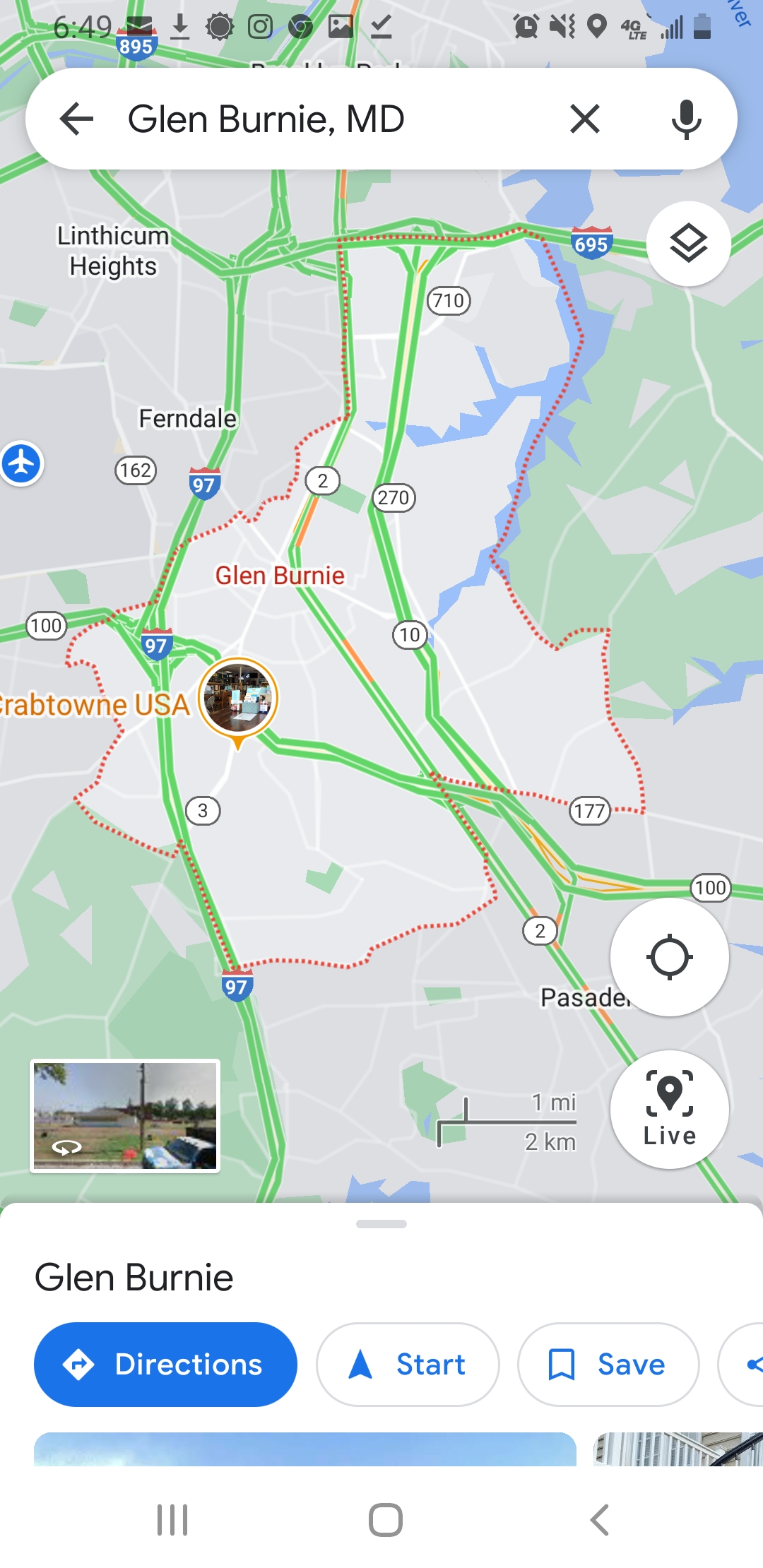The image is a detailed screenshot of a Google Maps app on a smartphone, showing a map and search results for Glen Burnie, MD. At the top of the screen, various phone status icons are visible, including the time "6:49," clock, Wi-Fi, and battery life indicators. Below these icons is a semi-elongated white search bar with the text "Glen Burnie, MD" in black letters. A series of navigational elements are highlighted on the map: green lines representing highways, with major highways marked by blue badges with red tops (such as Route 97), and smaller roads outlined in green (like Routes 710, 272, 10, 177, and 102). The area depicted is just north of Pasadena, featuring a mix of gray for built-up areas and green for open spaces. There's also a square box at the bottom with a real street view image of the highlighted location. Nearby, the words "Glen Burnie" reappear below the map, followed by a blue "Directions" button, a white "Start" button, and a round "Save" button. Additionally, on the lower section, there are two smaller circles: one for live location updates and another labeled "Live." The image also includes various navigation options and icons typical of a Samsung device, as well as multiple arrows and boxes indicating different features and functions of the Google Maps interface.